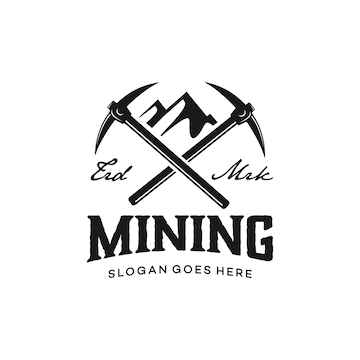The image is an illustrative logo template likely designed for a potential client's business. The logo is set against a white background and consists solely of black elements, embodying a minimalist and bold aesthetic. Central to the design are two crossed pickaxes, depicted with long, slender handles and sharp edges, forming an X shape with the left pickaxe overlapping the right. Above the intersection of the pickaxes, there is an outline of a mountain range featuring two peaks. Flanking the pickaxes on both the left and right sides is cursive text, difficult to decipher but possibly reading "END" or "ERD" on the left and "MERC" or "MRK" on the right, suggesting placeholder text. Below the crossed pickaxes, the word "MINING" is prominently displayed in large, bold, all-caps font, with a slight upward curve in its baseline. Beneath this, in a smaller, thinner all-caps font, the phrase "SLOGAN GOES HERE" is inscribed, indicating a customizable space for the company's tagline.